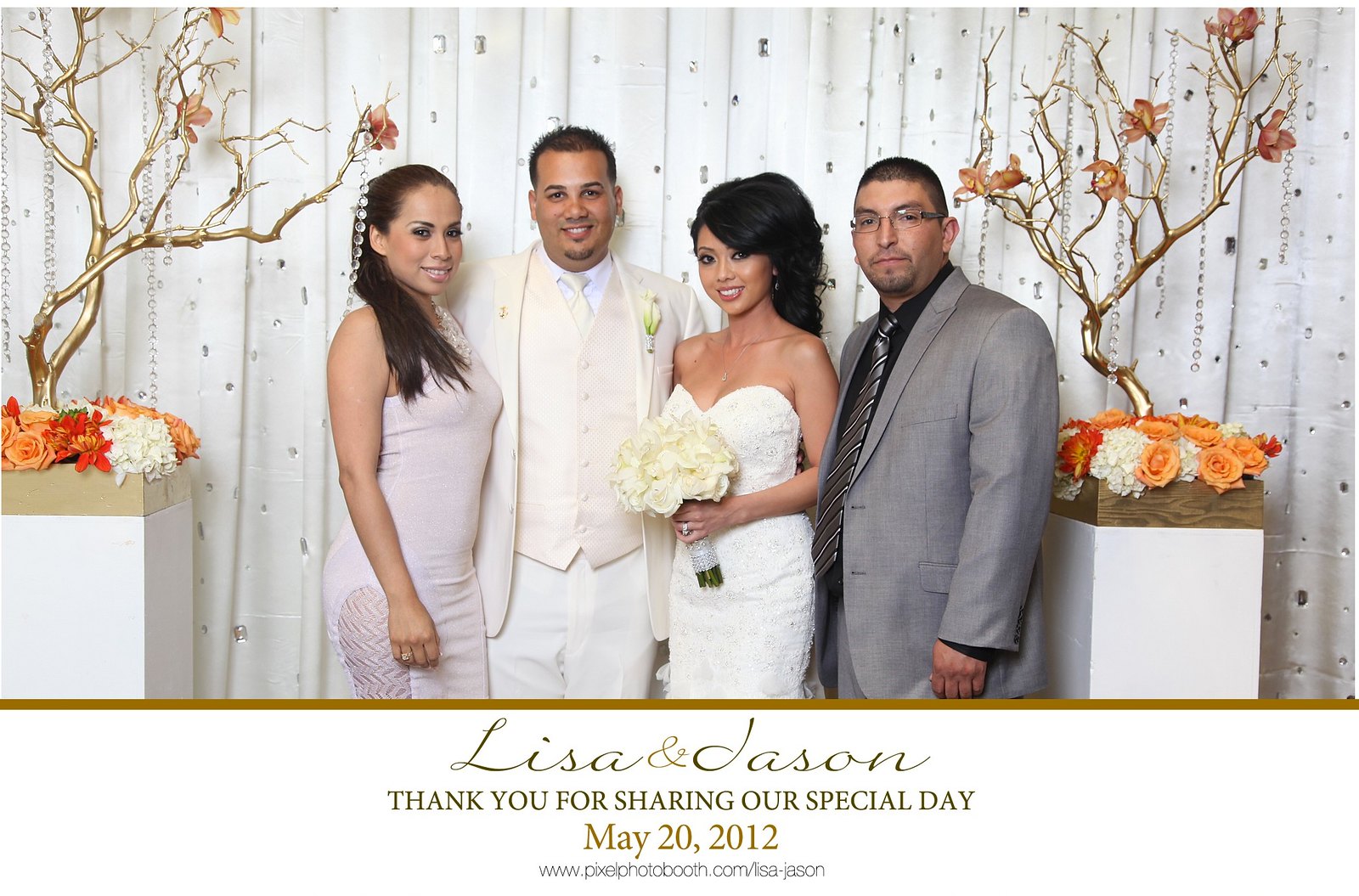In the photograph taken indoors, featuring a group of four people, the central focus is on the bride and groom, Lisa and Jason, celebrating their special day on May 20th, 2012. The image is framed by a decorative backdrop of white curtains with sparkling beads and flanked by pedestals adorned with golden tree branches and a mix of orange, white, and pink-toned flowers. 

From left to right, the first person is a woman with straight brown hair styled in a ponytail draped over her right shoulder, wearing a pale pink, sleeveless, form-fitting dress. Next to her stands the groom, Jason, dressed in a complete light-colored tuxedo with matching pants, vest, shirt, and a tie, his light brown skin complementing his short, spiky black hair. Beside Jason is the bride, Lisa, of Asian descent, with her dark black hair pulled back into a high ponytail. She is wearing a strapless white wedding dress embellished with lace and holds a bouquet of white roses. The fourth person is a man in a light silvery-gray suit with a matching striped tie and a black collared shirt.

At the bottom quarter of the six inches wide by four inches tall photo, a plain white footer displays a thin gold line, followed by the text in cursive, "Lisa and Jason," and in print, "Thank you for sharing our special day, May 20th, 2012," along with the URL, "www.pixelphotobooth.com/Lisa-Jason."